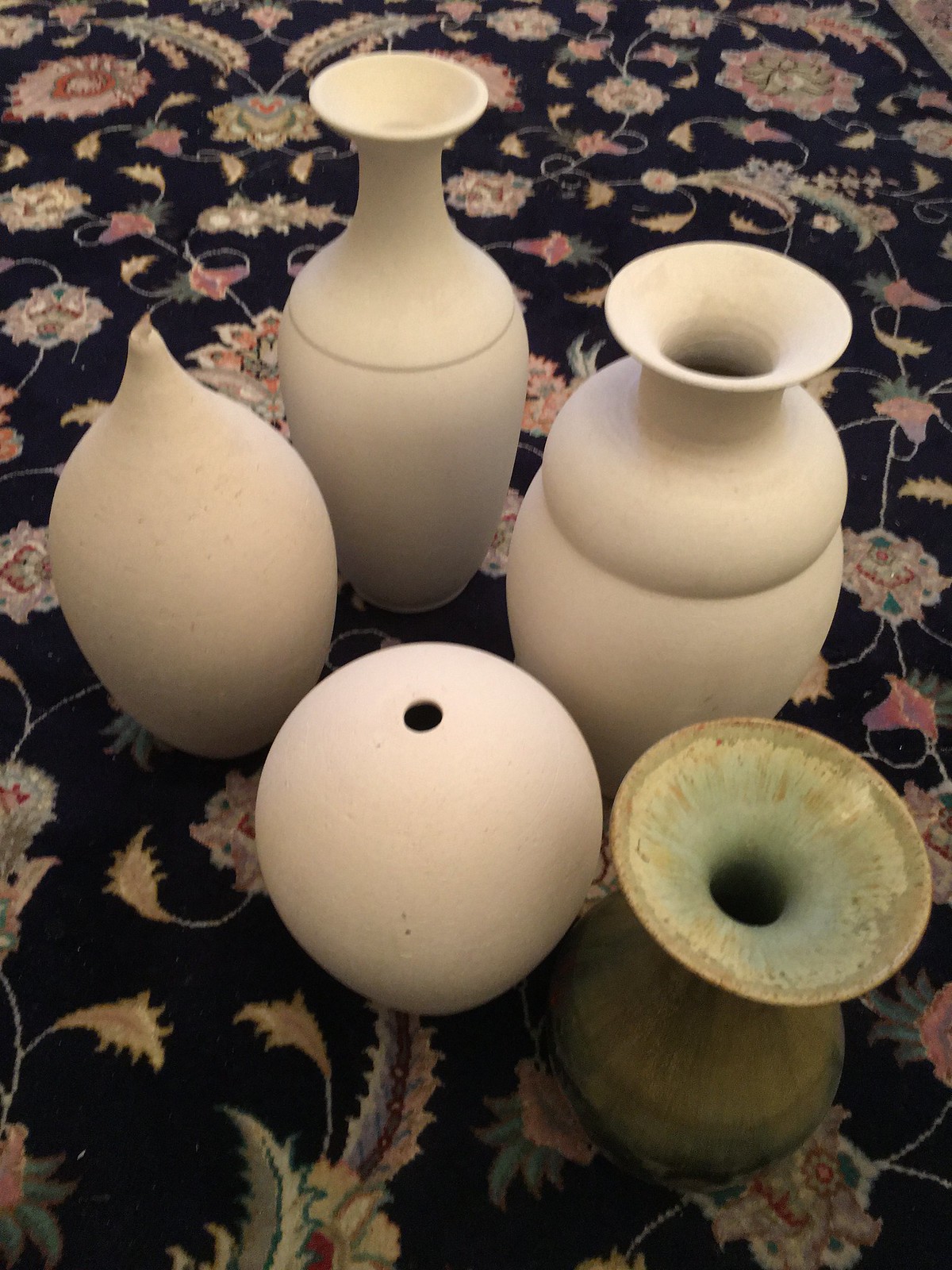This overhead image captures five distinct pieces of pottery resting on a black floral carpet. The intricate carpet features various flowers in pink, white, and yellow, interspersed with spiky green leaves. The pottery includes four white pieces and one greenish-blue piece with a rustic appearance and subtle wear, possibly indicating previous use. Each piece of pottery showcases a unique shape:

1. A spherical white piece with a hole in the center at the bottom left of the image.
2. A classic white vase in the middle, flaring out at the top with a pronounced lip.
3. A white piece to the top right with a complex design, featuring a rounded base, a constricted middle, and an outward flared neck.
4. A simple, small white rounded pot with a tiny tapered neck.
5. The distinctive greenish-blue piece on the right, with a narrow neck and a more pronounced, flared opening that has swirls of turquoise, yellow, and beige glazing. 

These pieces, likely handmade, exhibit varying neck widths and openings, indicating versatile potential uses, possibly as flower vases or decorative items.